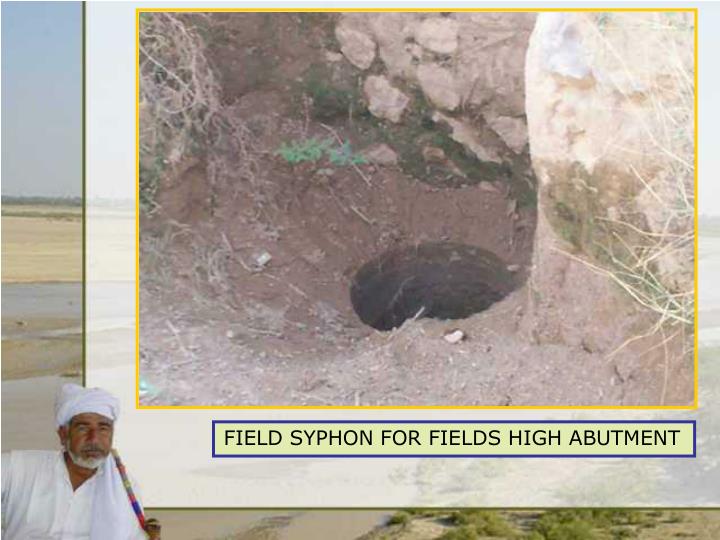The image prominently features a man standing in the bottom left corner, dressed entirely in white with a headdress or turban, and sporting white hair and a beard. He holds a colorful object featuring blue, red, yellow, green, and brown hues over his shoulder. In the background, a natural outdoor setting is evident, with a prairie or grassland landscape, some green shrubs, water, and rock elements. Positioned in the top right corner, a square inset displays a detailed, dirt-filled scene with a perfectly drilled hole at its center, surrounded by what appears to be dirt and roots or stems. Below this inset, black text on a blue rectangular background reads: “Field siphon for fields high abutment.” The entire inset image is bordered by a yellow frame. The colors in the image include multiple shades of yellow, blue, white, brown, green, black, and gray, suggesting the scene could be part of a presentation or an educational setting, possibly resembling a newspaper article.